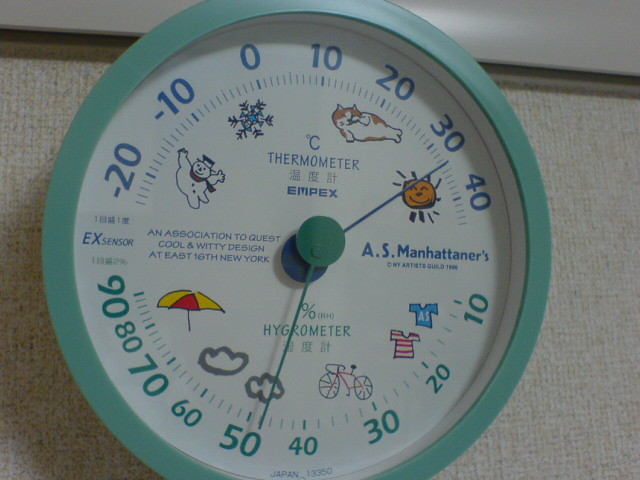Photograph of a Wall-Mounted Thermometer and Hygrometer by AS Manhattaners

This detailed photograph showcases a unique combination thermometer and hygrometer device mounted on what appears to be a wall with a fabric-like texture. The unit is designed by AS Manhattaners and prominently features a playful and witty design, reflecting its association with Quest Cool and Witty Design at East 16th New York.

The thermometer, positioned at the top, displays a temperature range from -20°C to over 40°C. The scale includes descriptive labels such as "Celsius thermometer" in English, accompanied by Chinese characters underneath, followed by the word "impacts." The thermometer is decorated with charming symbols: a Frosty the snowman at -20°C, a snowflake at 0°C, a resting cat at 20°C, and a sun at 40°C, indicating different temperature conditions visually.

Below the thermometer is the hygrometer, marked from 10% to 90% relative humidity. This gauge is adorned with various symbols as well, including an umbrella at 90%, clouds for intermediate humidities, bicycles suggesting favorable conditions, and a t-shirt symbol for low humidity, signifying comfortable weather.

The entire unit is enclosed in a turquoise rim, with a white central background for the measurement scales. The temperature readings are denoted in blue numbers, while the humidity levels are marked in green numbers, enhancing readability. This combination instrument not only provides practical information but also adds a touch of artistic flair to its surroundings.